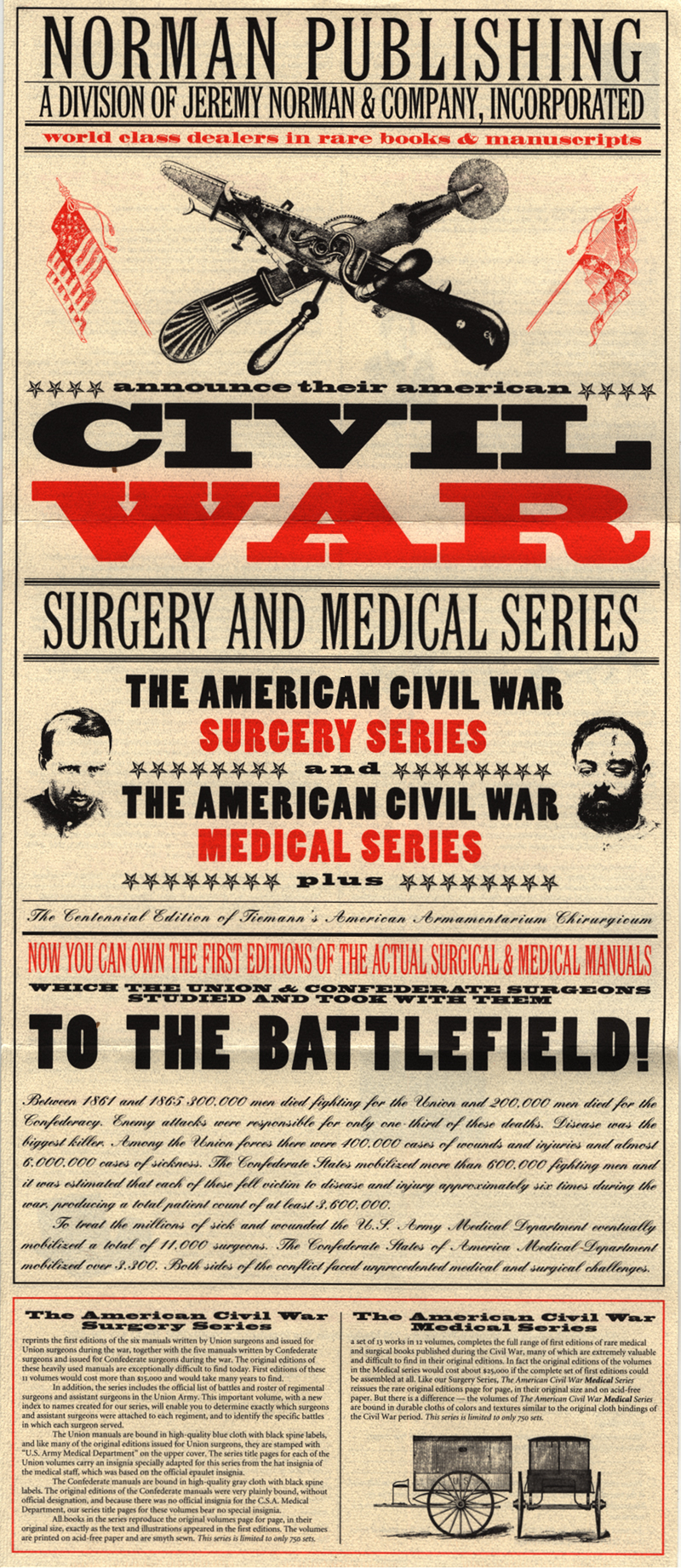The image depicts a vintage-looking, long rectangular poster with an off-white beige background adorned with black and red text. At the top, it prominently displays "Norman Publishing, a division of Jeremy Norman and Company Incorporated" followed by the tagline "world-class dealers in rare books and manuscripts" in small red letters. Below this text, crisscrossed are two old-style weapons, possibly knives. Adjacent to this imagery are flags, including an American flag, a Confederate flag, and possibly a British flag, each rendered in red. Centering the historical theme, the next section reads “Announces their American Civil War Surgery and Medical Series," listing both "The American Civil War Surgery Series" and "The American Civil War Medical Series."

The bulk of the poster contains detailed descriptions of these series, noting that they reprint the first editions of critical surgical and medical manuals used by Union and Confederate surgeons during the Civil War. It elaborates on the challenges faced by medical personnel of the time and includes statistical data on battlefield casualties and disease prevalence, emphasizing the severity of medical conditions during the war. The descriptions mention that the original editions of these manuals are rare and highly valuable, emphasizing that modern reprints are bound in durable cloths mimicking the styles of the Civil War period, either in high-quality blue for the Union or gray for the Confederacy.

Further down, the poster details the composition of the series, highlighting that it includes authentic reprints of 11 manuals for Union and Confederate surgeons, available in an exclusive set limited to 750 copies. It ends with a note on how these volumes are printed on acid-free paper, preserving the original size and illustrations. Illustrations include a drawing of a wagon viewed from the side and back, along with two portraits of gentlemen, reinforcing the historical and educational value of the reproduced manuals.